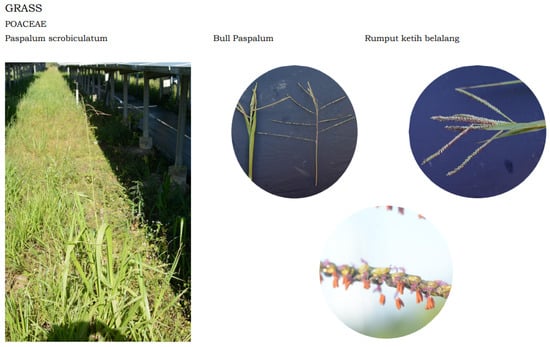The image is an infographic consisting of four photos that showcase different types of grass and their specific attributes. The main photo on the left is rectangular and depicts a long row of green, wispy grass basking in sunlight, with a blurred background that might include a wooden structure. Above this photo, it reads "Grass, Poaceae, Paspalum acrobiculatum."

To the right, there are three circular images arranged in a column. The two upper circles have blue backgrounds and feature close-ups of single blades of grass, each with seed pods at the top. The top-left circle details grass labeled as "Grass, Portia, Paspalum," while the top-right circle captions "Bull, Paspalum," with a focus on a brownish-tinged blade of grass. 

The bottom circle has a white background and shows a detailed close-up of grass seeds, the caption reading "Rupert Keith Beliching." This circle seems like a Petri dish and has small orange flowers at the end of the grass stalk. Overall, the image combines real-life grass photographs with detailed close-ups, along with scientific nomenclature and various visual backgrounds.